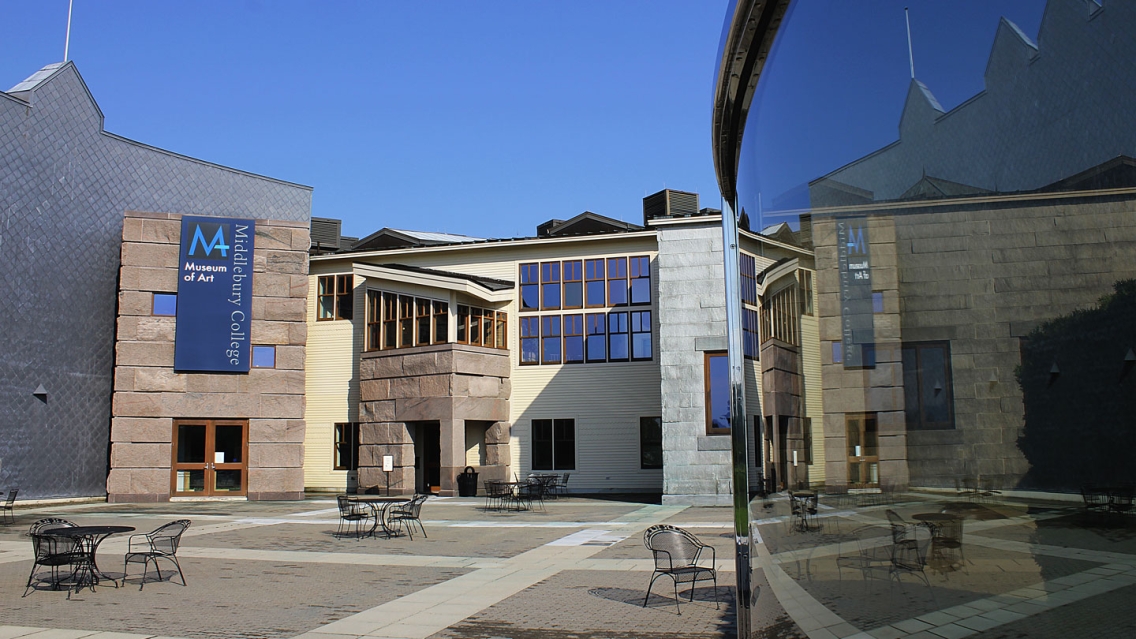This outdoor photograph showcases the exterior of various buildings surrounding an open plaza. At the center of the plaza, numerous round black tables with iron chairs are neatly arranged, each table typically paired with two chairs. Surrounding the courtyard are buildings of diverse architectural styles, featuring large stone blocks, sections of brown and white brick, and modern metal cladding. A prominent feature is the building on the right, adorned with a massive blue banner emblazoned with a large 'M' and labeled vertically as "Middlebury College" and horizontally as "Museum of Art" in white text. This building also features an extensive use of glass, including a distinctive curved glass structure that partially reflects the plaza. The floor of the courtyard combines light granite walkways with sections of brown bricks, and the scene is lit by a clear, cloudless blue sky, enhancing the vibrant and inviting atmosphere. Various signs are posted around the museum entrance, adding to the detailed and structured appearance of the space.